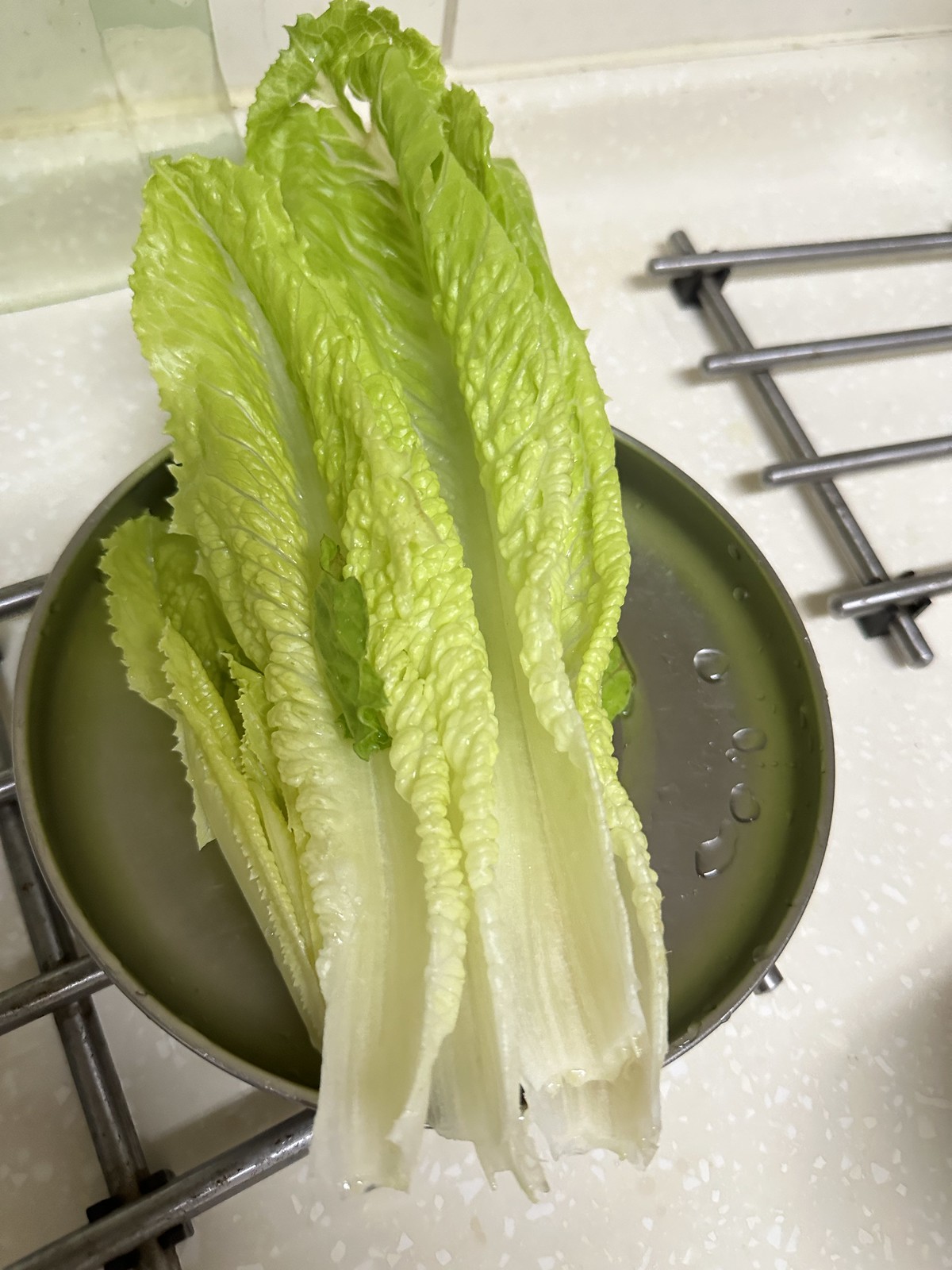This detailed, indoor photograph, taken in portrait orientation, showcases a food preparation scene centered on a light-colored or white countertop. At the heart of the image is a round, silver pan resting on a metal cross-beam structure with four prongs extending outward, resembling a hot plate setup. Placed on this pan are several freshly washed stalks of romaine lettuce. Each stalk is characterized by its long, white or cream-colored bases that transition into yellow and then bright green leaves as they flare out. Visible droplets of water or oil glisten on the lettuce and the interior right edge of the skillet, suggesting recent washing or preparation. In the upper right-hand corner, another silver gridded grate with four cross beams extends out of view, adding a touch of metallic contrast to the scene that features realistic elements of food photography.